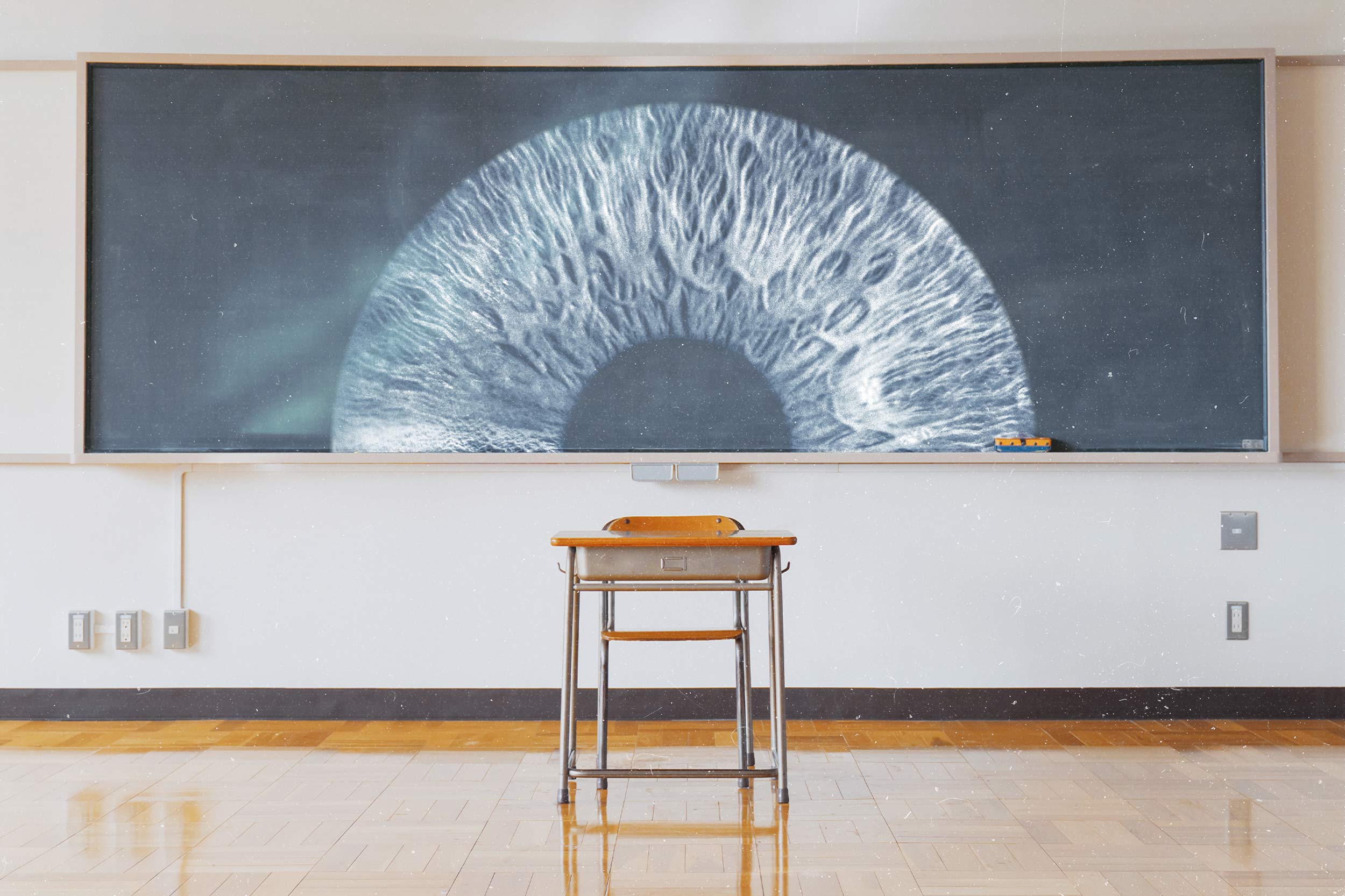This photorealistic image captures the interior of a seemingly empty classroom. Central to the image is a single, old-style student desk, its light orangey-brown wooden surface complementing the shiny light brown wooden floor beneath it. The desk, complete with a silver metal frame and an attached chair facing the camera, sits directly in front of a large, black chalkboard. The chalkboard, edged with a white border, dominates the white wall behind it. Intricately sketched in white chalk on the blackboard is a highly detailed, close-up drawing of the top half of an iris, with the fibers and pupil clearly defined. The drawing is positioned so that the desk aligns with the bottom half of the pupil, emphasizing the meticulous artistry involved. The overall emptiness of the room, coupled with the focused, striking artwork, creates an intriguing and contemplative atmosphere.